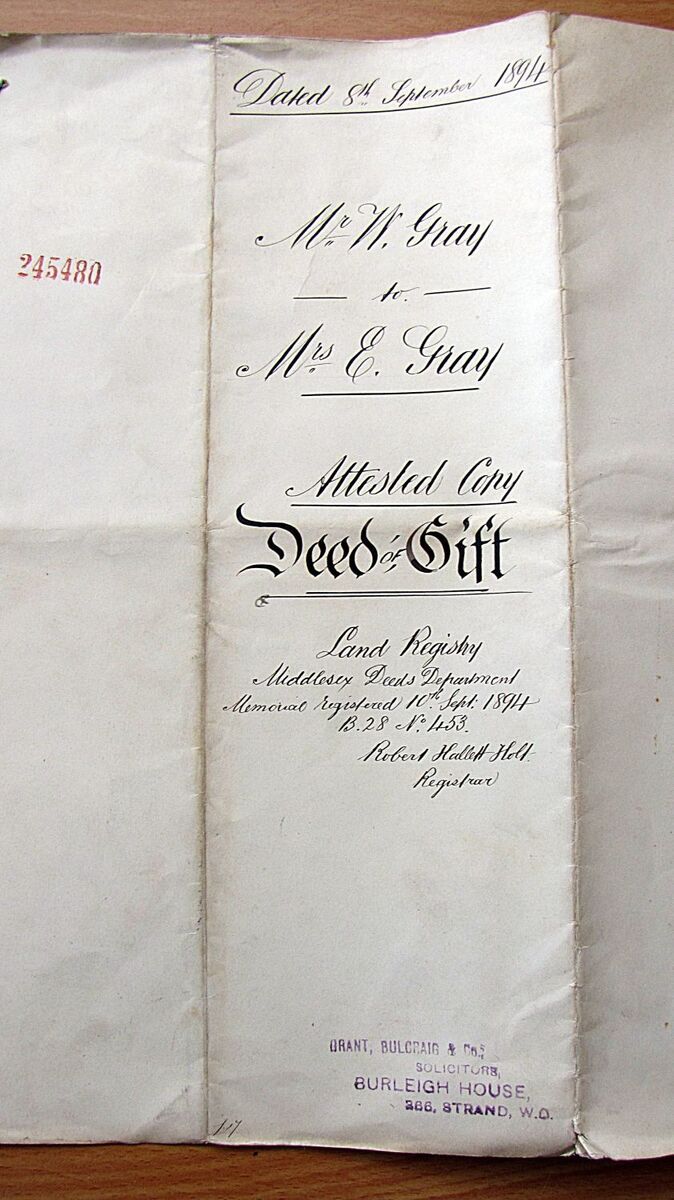This image depicts a historic Land Deed document dated 8th September 1894. At the top, written in elegant black cursive, is the date, followed by a line underneath. Below the line, the document lists "Mr. W. Gray," then "to Mrs. E. Gray," indicating the transfer of ownership. In a distinguished older font, it prominently features the title "Deed of Gift." Further down, it references the Land Registry, specifically the Middlesex Deeds Department, with additional details noting the Memorial Registered on the 10th of a certain month in 1894, cataloged as B-28, number 1053. The registrar is noted as Robert Hethfield Hell, although the handwriting there is challenging to decipher. Towards the bottom of the document, a purple ink stamp reads "Grant Bull Crane and Company, Burr Lye House, 266 Strand, W.O." The document also includes an additional red stamp marked "245 480," which might be on an adjacent page.